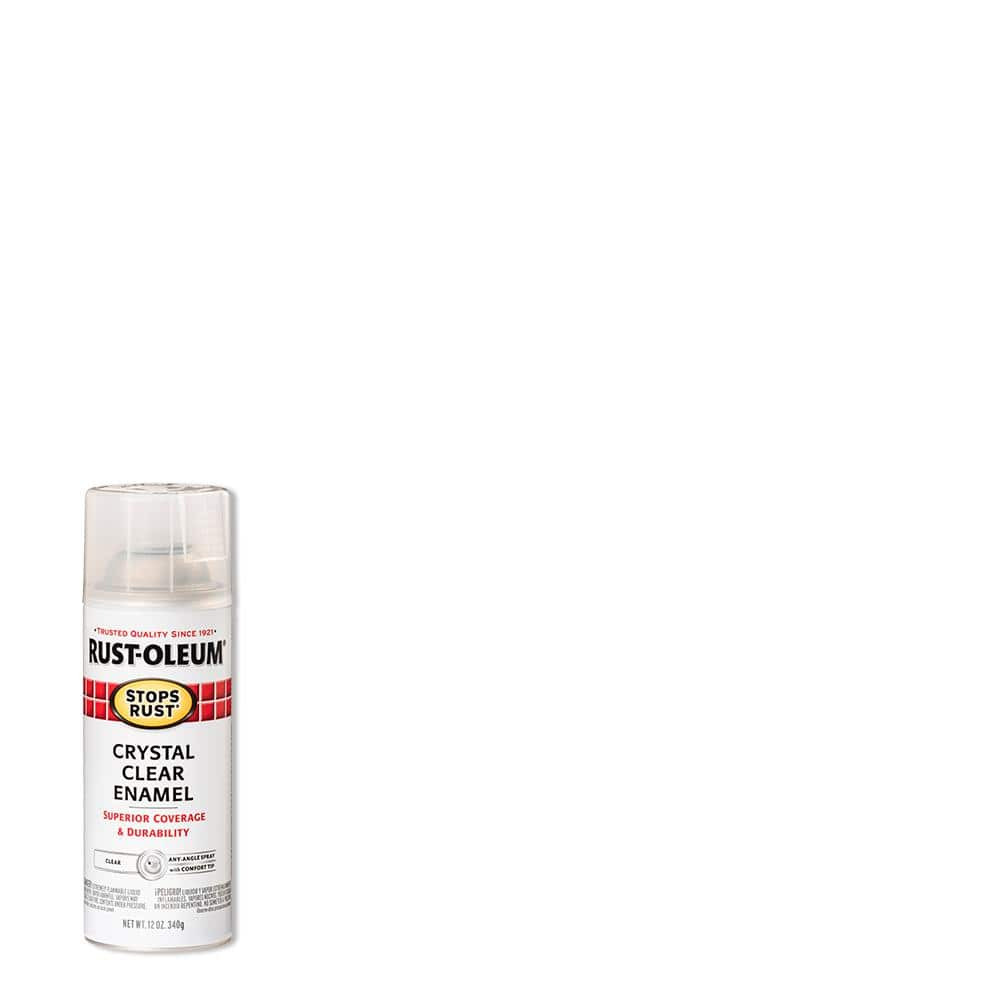This is a highly detailed photograph of a can of Rust-Oleum spray paint, prominently labeled "Trusted Quality Since 1921." The white can features a translucent white cap and a metallic, curved top with a comfort tip for any-angle spraying. Dominating the design is the text "Rust-Oleum" in bold black print. The slogan "Stops Rust" is prominently displayed in black letters encased in a yellow oval, set against a backdrop of red square tiles. Additional text includes "Crystal Clear Enamel," emphasizing superior coverage and durability, written in black capital letters beneath the logo. Below, in smaller red font, is another mention of the superior coverage and durability. The overall weight is specified as 12 ounces (340 grams), and fine print can be seen at the bottom of the can. The product is designed to provide clear protective enamel with longevity and resistance against rust. The can is set against a plain white background, focusing attention entirely on the product.